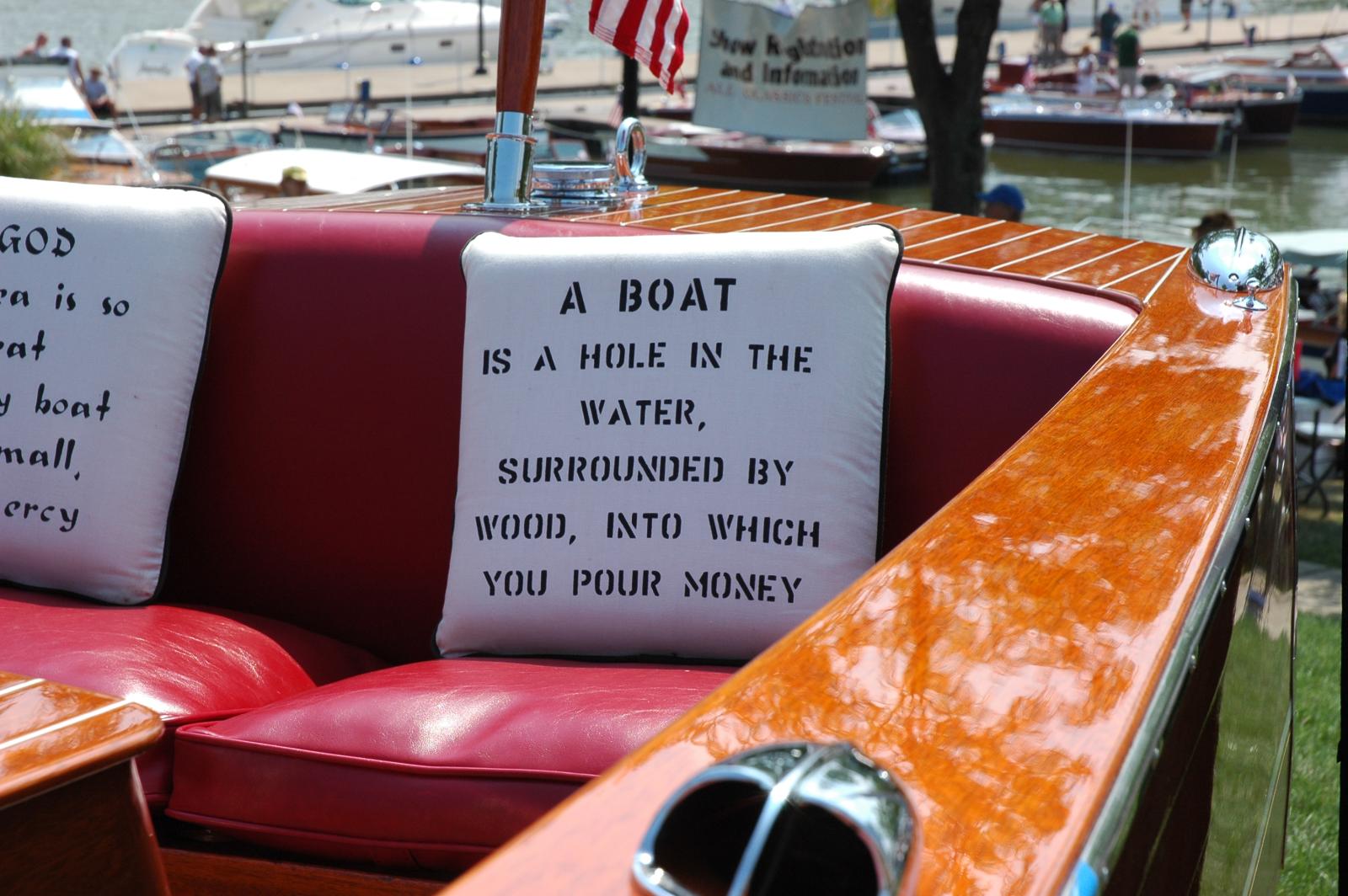In this daylight photograph set outdoors on the water, the focus is on the back area of a glossy, wooden boat with a rich reddish-brown frame. The boat is moored at a dock, with an American flag mounted on a pole at the rear edge of the boat, glimpsed even from a partial view. The seating area features plush, red leather cushions with wooden rails that display a polished sheen under the sunlight. Two white pillows rest on these seats: the visible one on the right bears the saying, "A boat is a hole in the water surrounded by wood into which you pour money," in black stenciled letters. The left pillow is partially obscured, with only fragments of its text showing. In the background, the setting includes a lively dock area with boats. Behind the boat, a boardwalk populated with strolling people is visible, along with a banner announcing "show registration and information." The sun casts a warm glow over the entire scene, illuminating the details of this charming maritime tableau.